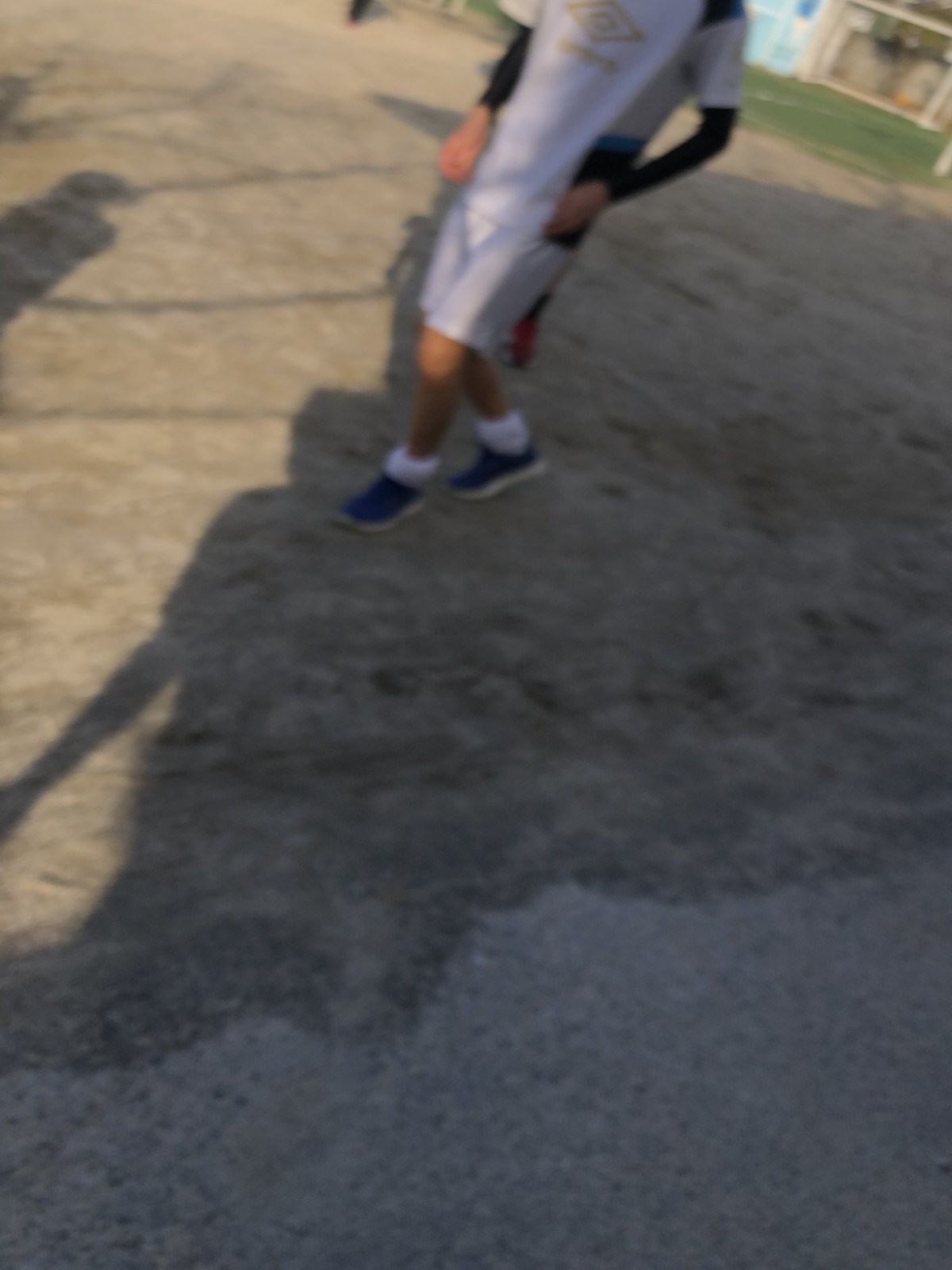This blurry photograph captures a male individual walking on an area that might be a mix of light gray-blacktop and discolored dirt, with hints of a potentially dead athletic field in the background. The individual is dressed in long gray shorts, blue sneakers, and white socks bunched down at the ankles. He's also wearing a white t-shirt with a gold diamond-shaped logo at the center, layered over a long-sleeve black shirt. The image is shadowy with parts highlighted by sunlight in the top left corner, revealing another figure in shadow and the edge of a house with a grassy front yard. The scene features items like poles hinting at soccer goals and white chalk marks on the ground, suggesting an athletic setting. Rectangular shadow shapes are also visible on the left side, adding to the photograph's depth.